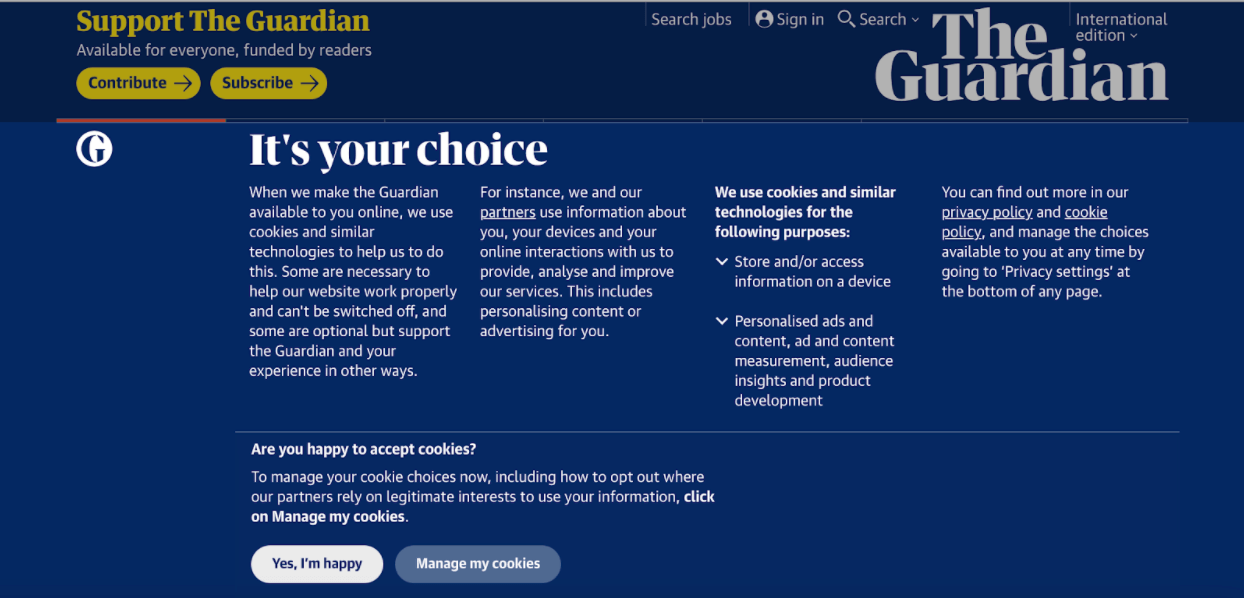A detailed description of the image is as follows:

The image is a left-to-right horizontal screenshot from a web page that can be accessed from either a computer or a smart device. At the top, there is a dark blue rectangular banner stretching from left to right. In the upper left-hand corner of this banner, a yellow text reads, "Support the Guardian." Below that, in white text, there is a message saying, "Available for Everyone, Funded by Readers." Adjacent to this message are two yellow buttons: one labeled "Contribute" and the other "Subscribe," both featuring arrows pointing to the right.

Towards the right side of this top banner, there is a collection of navigational elements, including a text link for "Search Jobs," a sign-in button, and a search function symbolized by a magnifying glass icon. Further to the right, the words "The Guardian" are displayed in white next to "International Edition."

Below this dark blue banner is a slightly lighter blue section. In the upper left corner of this area, an icon resembling the letter "G" is displayed. Adjacent to it is a bold white headline stating, "It's Your Choice." Under this headline, a paragraph details the use of cookies on the website, explaining that some cookies are necessary for the website's functionality while others enhance user experience.

The paragraph continues to elaborate on the purposes of these cookies, separated by a thin gray line at the bottom of the text. Below this divider, there's a question asking, "Are you happy to accept cookies?" followed by two clickable options: "Yes, I'm happy" and "Manage my cookies."